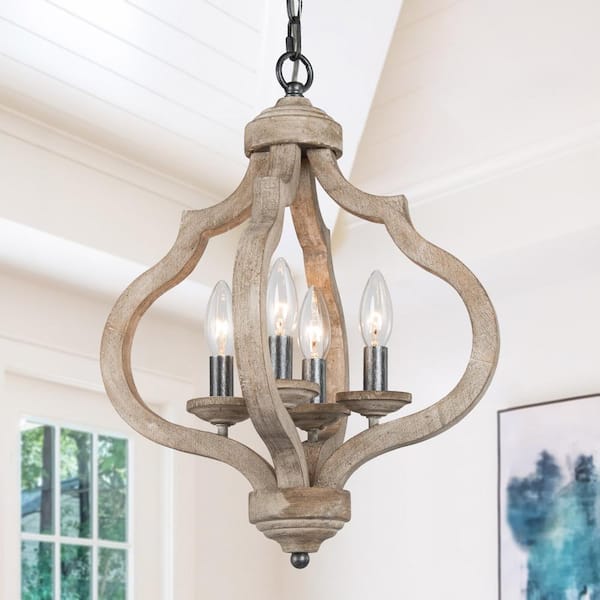The photograph showcases a beautifully detailed indoor scene dominated by a striking wooden chandelier with a farmhouse aesthetic. The chandelier, suspended from the ceiling by a black chain, features a rustic design with four elongated bulbs arranged in a bell-like structure, each piece of wood connected by a circular wooden base. The setting is an immaculate, white-painted room with a shiplap vaulted ceiling, exuding a blend of contemporary cleanliness and traditional warmth. In the background, to the bottom left, there is a doorway fitted with six rectangular window panes framed by pristine white wood, suggesting an entrance or an exterior door. To the bottom right, part of a framed artwork is visible; it has a minimalist aesthetic with blue watercolor splotches on a white background. The overall ambience of the room is bright, open, and spacious, lending itself an almost surreal, possibly AI-generated quality due to the pristine and slightly blurred appearance.